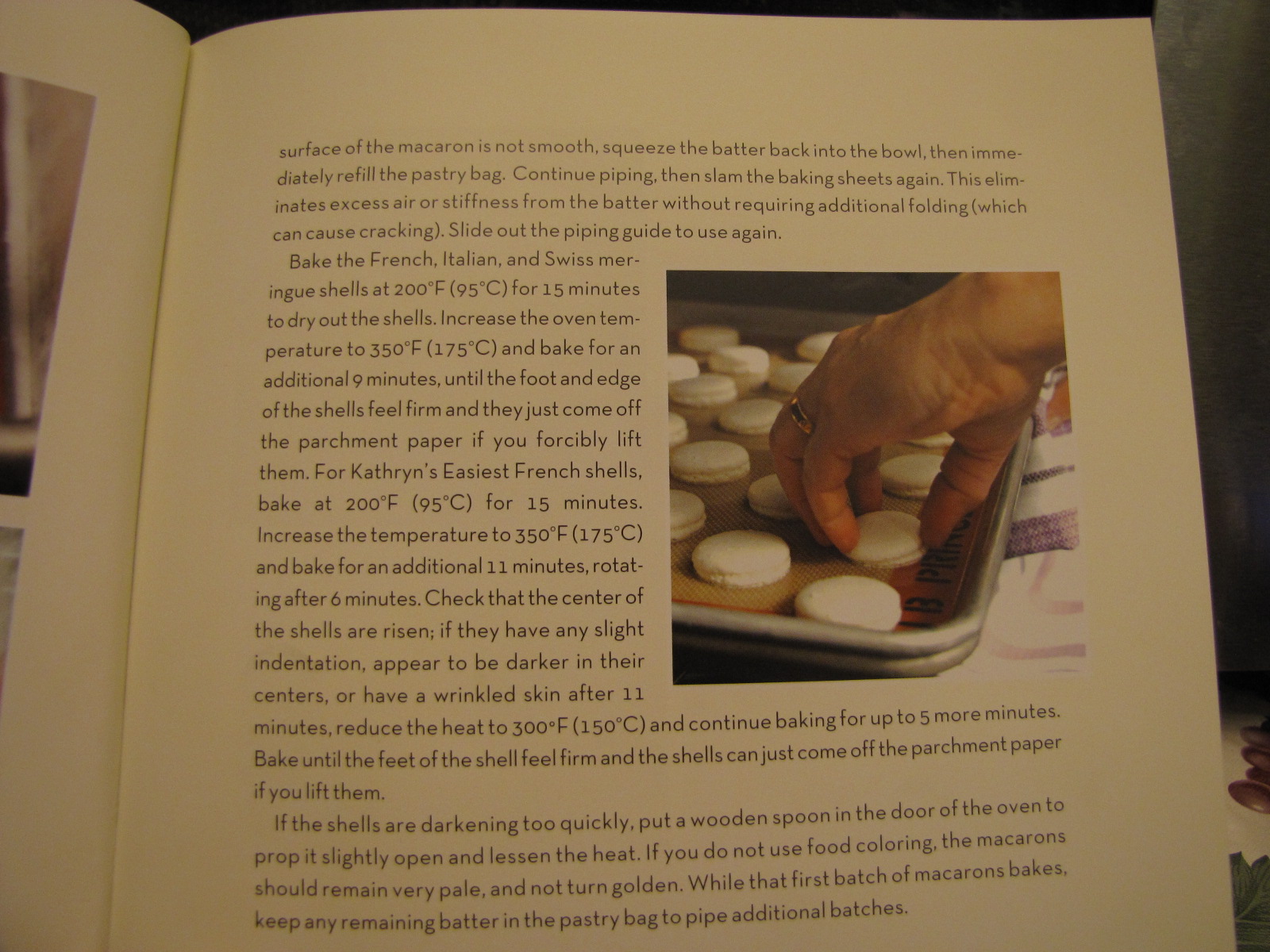The image is a horizontal rectangular photograph of an open cookbook, positioned flat on a dark background, likely a desk or table. The focus is on the right-hand page, which features a detailed, black text on a white background, laid out in a clear, readable font. This page includes a descriptive passage about different meringue techniques—mentioning French, Italian, and Swiss versions—providing both cultural context and instructions within narrative paragraphs rather than a list format. Prominently displayed is a photograph of a hand placing meringues or macaroons on a parchment-lined cookie sheet, showing an orderly arrangement of the white confections. The left-hand page is partially visible, revealing some additional text and an unclear image. This older-looking page has slightly yellowed paper and smaller text, adding to the overall sense of a well-used and informative cookbook.